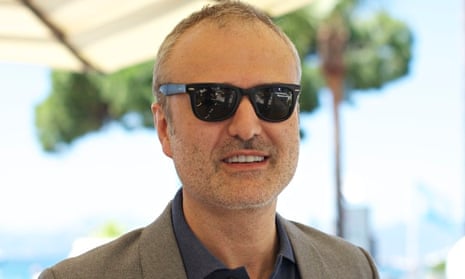The photograph captures a close-up of a middle-aged, light-skinned man with sunglasses, taken outdoors on a bright, clear day. He is smiling, revealing his top row of white teeth, and has a five o'clock shadow with stubble slightly darker around the mustache area. His very short hair and beard have a light grayish tone with a hint of brown, and he has a receding hairline. He wears a dark blue collared shirt under a gray or beige business jacket. The background is blurry and indistinct, featuring a bright sky, some greenery likely from a tree, and an overhead structure that appears to give him shade, possibly a cream-colored umbrella or awning supported by a thin brown framework. Additional indistinct shapes in the background suggest buildings, blue and white objects, and a brown post to the right of his head.